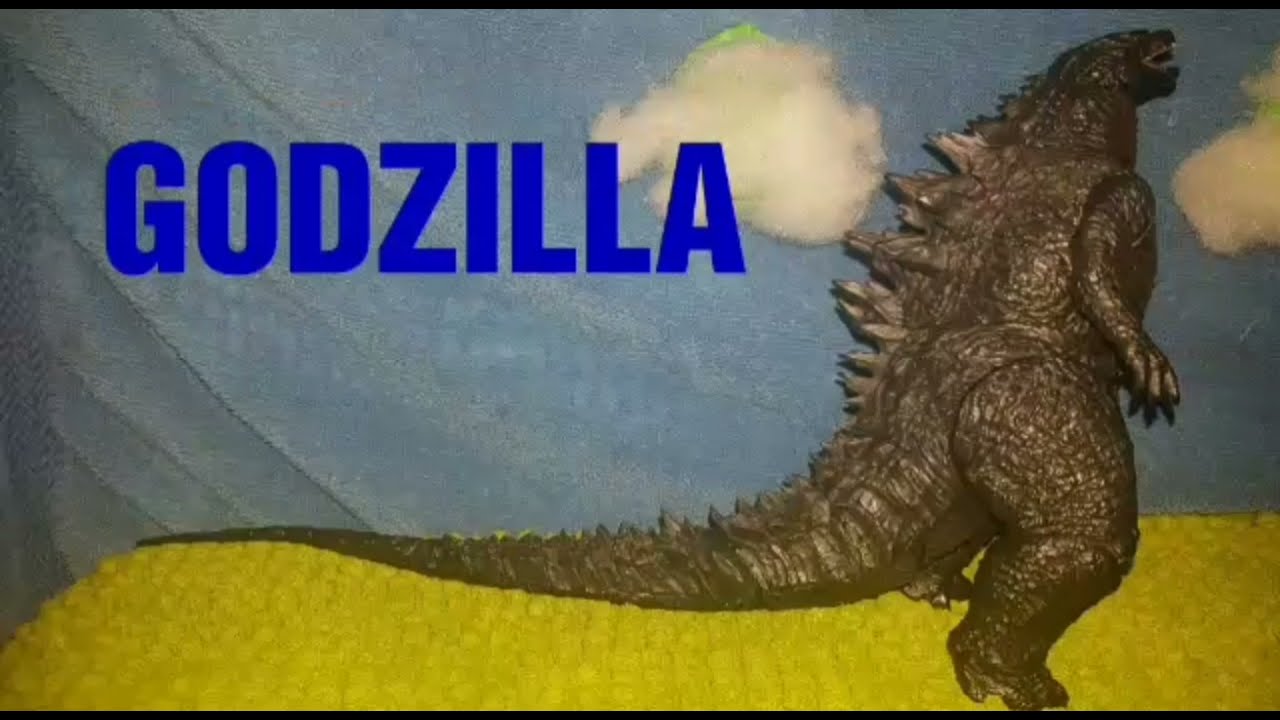This horizontal rectangular image, framed by thin black borders at the top and bottom, appears to be a scene featuring a Godzilla action figure in a homemade setting. The background mimics an outdoor sky, created with a light blue blanket adorned with white, cotton ball clouds. Set on a yellowish-green surface, which resembles a rug, the Godzilla figure dominates the right side of the image. The toy is depicted in a mostly dark black color, with some brownish-gray undertones, and features large spikes on its back. Godzilla, standing upright with his arms extended forward and mouth agape, appears to be looking towards the upper right corner. His long tail sweeps across the bottom of the frame towards the left. The scene is illuminated with indoor lighting. Enhancing the thematic effect, the word "GODZILLA" is prominently displayed in bright blue, all-capital letters across the upper left portion of the image, stretching towards the figure. This detailed setup evokes the impression of a still frame from a homemade movie, thoughtfully constructed to highlight the iconic monster.